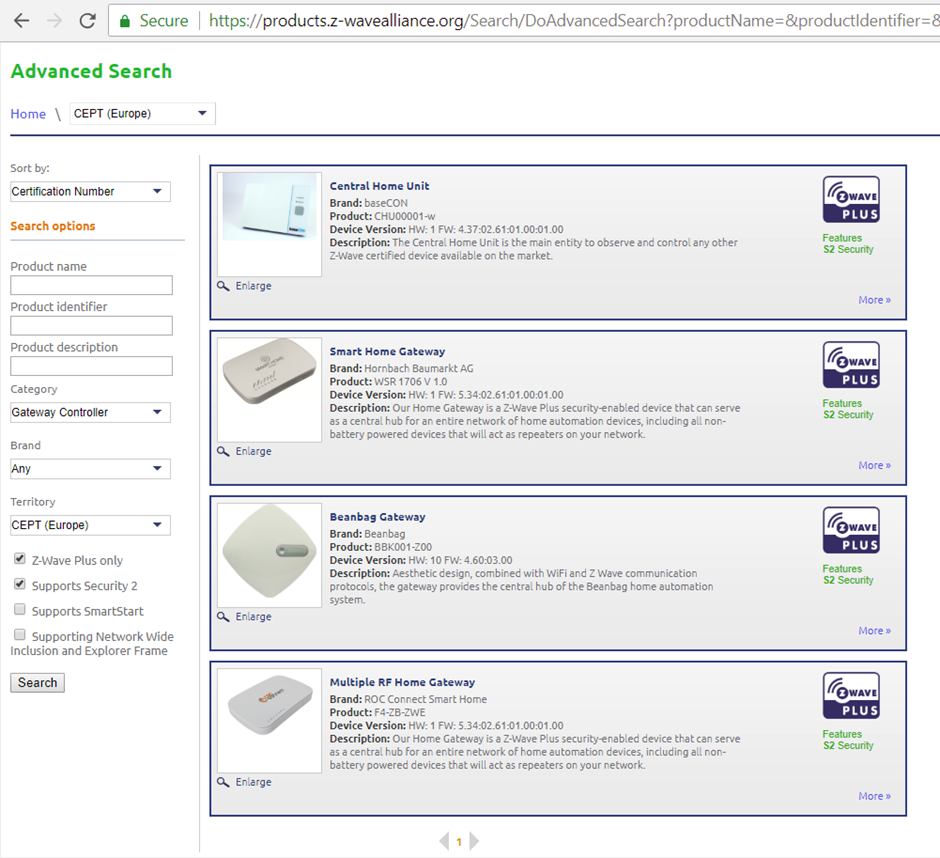This image appears to be a screenshot of a highly detailed advanced search page on a secure HTTPS website, specifically at the URL "products.z-wavelines.org." The page features various search and filter options for home safety products available in Europe. 

The search form comprises fields for entering a product name, product identifier, product description, category, brand, and territory. It also includes options to sort results by certification number. The user can filter products based on specifications such as Z-Wave Plus, Security 2 support, SmartStart support, Network-Wide Inclusion, and Explorer Frame support. 

Detailed icons and interactive elements are laid out in a grid of grey squares, alongside central command buttons like "Search." There is an emphasis on Z-Wave Plus features, showcasing various brands and central home unit capabilities, such as the "SmartHomeGateway HornBog," with identifiers like "Bog1 IG AWSR 1706 V1.0." Features listed include support for Z-Wave Plus security, central hub functionalities, network support, and a mention of Matter network compatibility. Other notable items in the layout include mentions of products like "BeanBag Gateway" and "BeanBag Multiplier Home Gateway RLC Connect SmartHome."